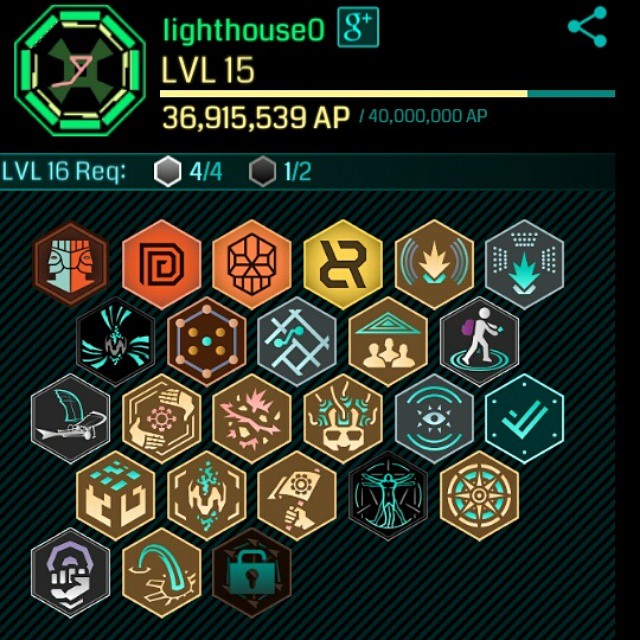This image is a screenshot taken from an old video game, titled "Lighthouse Zero," presumably the username of the player. The game interface suggests a talent system or skill tree, prominently displayed on a light teal background with black and blue diagonal stripes. The player's level is indicated as LVL 15, along with an achievement points (AP) count of 36,915,539 out of 40,000,000 required for the next level. 

The diagram consists of five rows of different colored pentagon and octagon shapes, each containing unique symbols. These symbols include an orange and black motif, and various other colors such as yellow, gold, black, brown, turquoise, and cream. 

The symbols depict a variety of images: an eye emitting blue waves, a man with wires going into his brain, a pair of hands turning a wheel, a nuclear explosion, and a dragon, among others. There are also more specific icons like a plane, a star, a blue typhoon, a blue explosion, a blue portal, a man standing over a portal, multiple people, double blue check marks, a skull, a crown, a letter D, a fist punching a circle, and diagrams of Vesuvius Man. 

The top right corner includes an outdated Google Plus link, emphasizing the image's age. The AP tracking points to requirements for leveling up, noted as "4-4" and "1-2" next to more small octagon shapes.